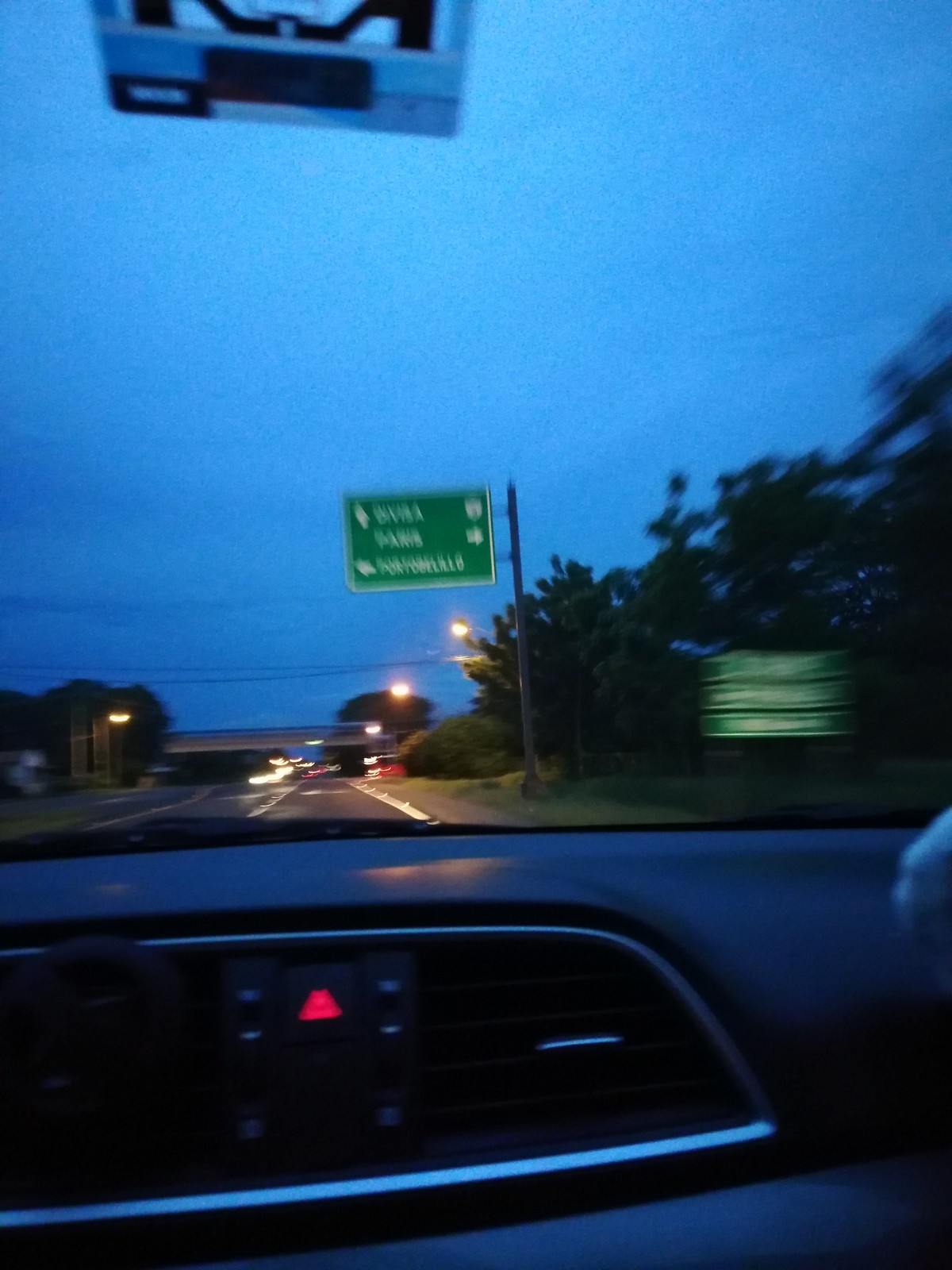The image showcases an interior view of a car's dashboard at night, with a blue-tinged evening sky visible through the windshield. The dashboard, featuring plastic components with silver lining and faux leather, displays a prominent red hazard triangle. Outside, the scene ahead is illuminated by multiple streetlights atop lamp posts and punctuated by white headlights from oncoming traffic. The left side of the road reveals black asphalt and approaching vehicles, while the right side shows blurry green grass and possibly some forest area. Overhead, a green interstate sign with blurry text indicates directions, suggesting destinations like Paris and Porto Belilo. Adjacent to this sign, electrical lines are visible against the sky. The road appears to be a busy city highway, further hinted by a crosswalk or overpass in the distance—a setting that's transitioning between dusk and full nightfall.